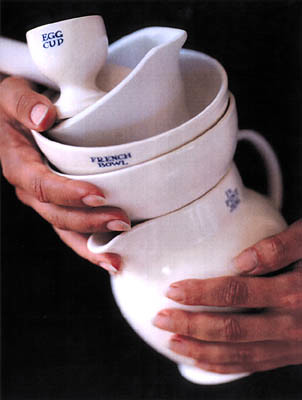This close-up photograph captures a dark-skinned woman’s hands, adorned with slightly dirty pinkish nails, holding a meticulously stacked collection of ceramics against a solid black background. At the base is a white pitcher, featuring blue inscriptions that are unclear. Nested atop the pitcher are two bowls—the outer one plain white and the inner one labeled "French Bowl" in blue letters. Sitting within the "French Bowl" is a small vessel resembling a mortar or a gravy dish with a spout, also in white. Crowning this stack is a delicate egg cup, marked with the words "Egg Cup" in blue. The composition emphasizes the contrast between the ceramic whites and the model’s dark skin, further highlighted by the deep black backdrop.